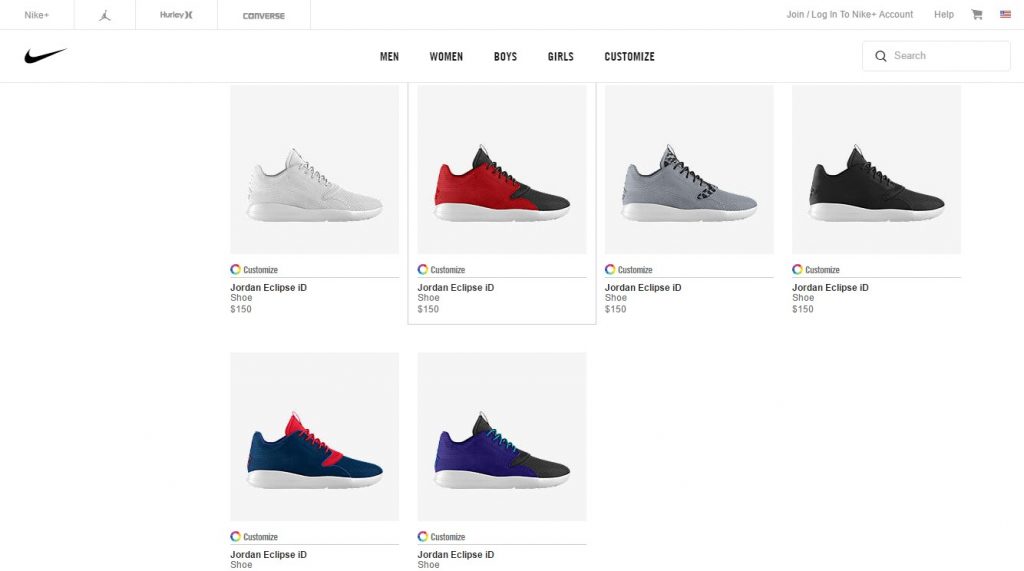The screenshot displays a webpage primarily featuring a selection of Nike products. Prominently visible at the top are the logos for Nike, Air Jordan, Hurley, and Converse, alongside a plus symbol indicating the Nike+ loyalty program. The navigation bar includes options to join or log in to a Nike+ account, access help, view the shopping cart, and select the American flag for the United States region. Categories for browsing products such as Men, Women, Boys, Girls, and Customized are displayed in a box next to a search function.

The main content area showcases two rows of shoes. In the first row, there are four pairs: the first pair is white, the second pair features a red and black design, the third pair is gray, and the fourth pair is black. In the second row, there is a pair of predominantly blue shoes with a greenish-blue tint and hints of red and black accents.

Each shoe has an option labeled "Customized" beneath it, and next to this label is a circular icon divided into three sections colored red, yellow, and green.